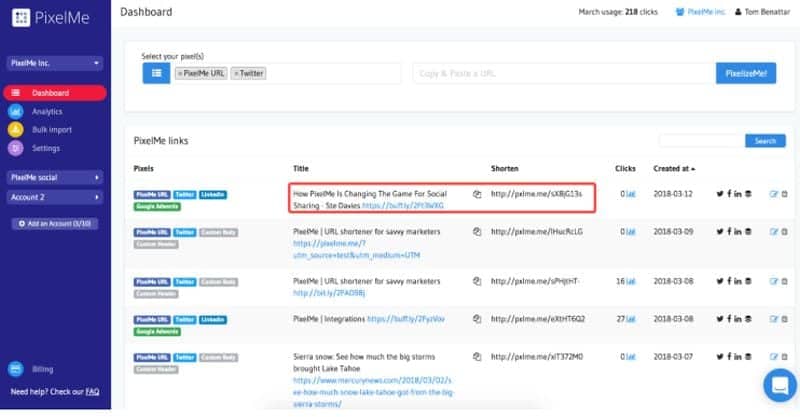Screenshot of a "Pixie Me" Dashboard

This detailed screenshot captures the interface of a "Pixie Me" dashboard. The layout features a blue vertical sidebar on the left with several navigation elements: a "Dashboard" section, a search bar, a blue button labeled "Analytics," a yellow button for "Bulk Import," and a purple circle icon for "Settings." The central portion of the dashboard displays numerous components seemingly related to "Pixie Me Links."

At the top of the main section, two search bars are prominently placed for easy access. Below these search bars, there are four blue buttons, whose exact functions are somewhat blurry but relevant to operational tasks. The core of the dashboard displays a grid layout containing various metrics and controls including "Pixies," "Title," "Shorten," and "Click."

Additionally, the interface includes social media integration with icons for Twitter, Facebook, and LinkedIn among others, although these are fuzzy and hard to decipher. The main content appears organized into four distinct rows, each populated with different links and associated data.